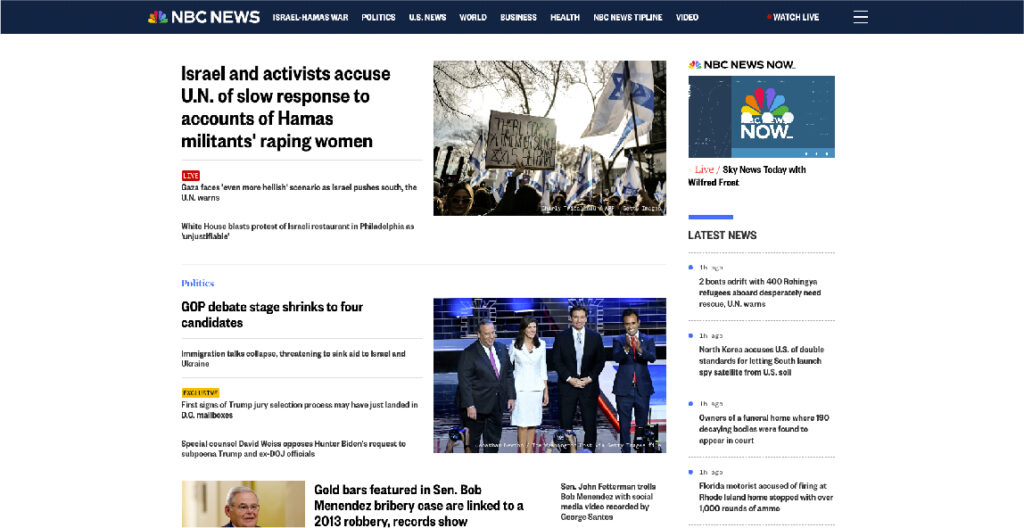The homepage of the NBC News website displays various news categories such as Politics, U.S. News, World News, Business News, and Health News. Prominently featured is coverage on the Israeli-Hamas conflict, with a headline that reads "Israel and Activists Accuse UN of Slow Response to Reports of Hamas Militants Raping Women." Adjacent to this main story are two more related articles and a photograph showing protestors holding the Israeli flag, likely in opposition to Hamas.

Further down, the Politics section presents updates on the Republican presidential nominees, spotlighting figures like Ron DeSantis alongside three other candidates, and a headline states "GOP Debate Stage Shrinks to Four Candidates." Additionally, there’s an article featuring Senator Bob Menendez, with the headline "Goldbar Featured in Senator Bob Menendez’s Bribery Case Linked to a 2013 Robbery, Records Show." Below these sections are links to the latest news articles, providing a comprehensive overview of current events and political developments.